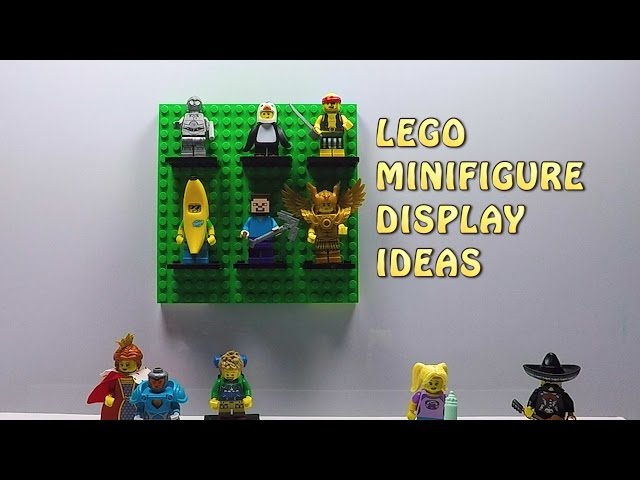The image showcases a vibrant and detailed scene of various Lego minifigures arranged for display purposes. The backdrop features a gray wall framed by a black border, creating a contrast that highlights the colorful characters. Anchored to this setup is a green Lego piece with two rows of three shelves each, holding minifigures. The top row houses a gold, robotic C-3PO-like figure with wings, a figure in a penguin costume, and a pirate. The bottom row consists of a minifigure in a banana suit, a Minecraft character, and a figure resembling Loki from the Marvel universe.

Below this organized display, on a white surface, sits a collection of additional minifigures. Among them is a character wearing a sombrero, a woman with blonde hair, and others dressed in various costumes, including one holding a small trophy that resembles the Stanley Cup. On the right side of the image, bold yellow text in capital letters reads "LEGO MINIFIGURE DISPLAY IDEAS," suggesting the image is likely a still from a YouTube video or similar content aimed at providing viewers with creative ways to showcase their Lego minifigure collections.